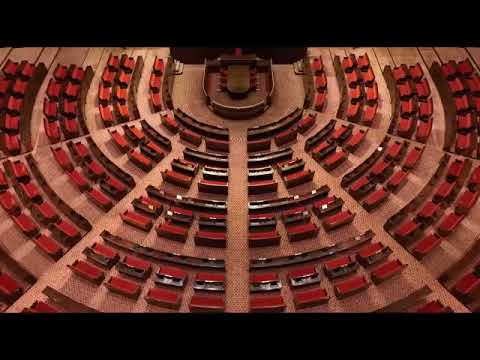This image captures an elevated, almost bird's-eye view of a circular amphitheater, taken from about 50 feet above, possibly from a high balcony or suspended from a ceiling. The amphitheater's seating area is arranged in a semicircular formation with rows of red chairs, each row consisting of two sub-rows separated by a blank space. This seating pattern gives the appearance of a letter "U" from this vantage point. The chairs seem to have brown or black barriers separating the groups, and each seat has a red foam cushion with a brown backing. The circular sectors of the seating area are divided by aisles that create a clear path through the rows. In the center of the amphitheater is a stage with a platform surrounded by walls, resembling the shape of a shield. The image is framed by plain black rectangular strips at the top and bottom, adding a stark contrast to the detailed interior view of the amphitheater that almost appears computer-generated due to its clarity and precision.